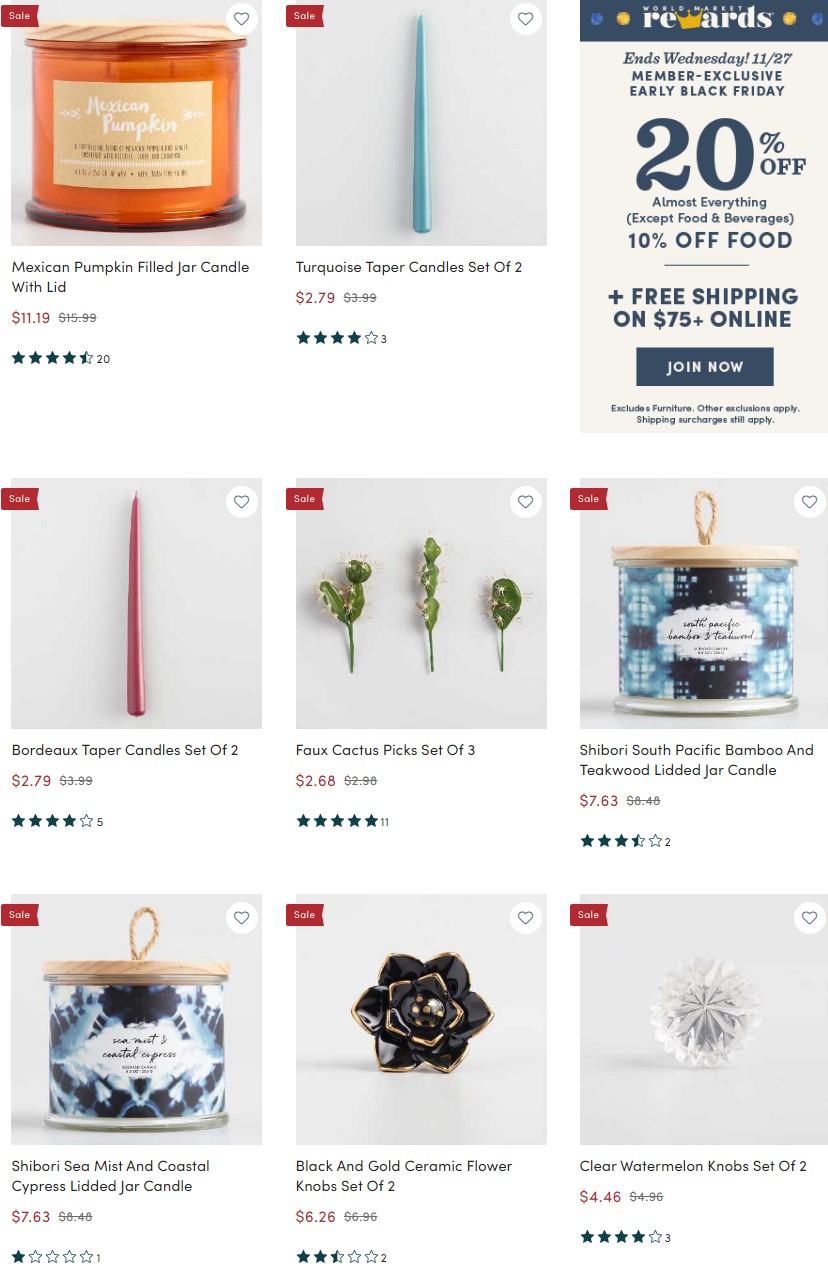This image is a detailed screenshot of an e-commerce website showcasing a variety of items for sale. At the top of the site, there are two main products featured: on the left is a Mexican Pumpkin Filled Jar Candle with Lid, priced at $11.19, and on the right is a Turquoise Tapered Candle Set of Two, available for $2.79. 

In the upper right corner of the screen, a promotional banner advertises a sale offering 20% off almost everything except food and beverages, 10% off food, and free shipping on orders over $75.

Moving to the center row of items, starting from the left, there is a Bordeaux Tapered Candle Set of Two for $2.79, followed by a Faux Cactus Picks Set of Three, priced at $2.68. Next is a Shibori South Pacific Bamboo and Teak Wood Lidded Jar Candle for $7.63.

In the final row, the items displayed are: a Shibori Sea Mist and Coastal Cypress Lidded Jar Candle for $7.63, a Black and Gold Ceramic Flower Knob Set of Two for $6.26, and a Clear Watermelon Knob Set of Two priced at $4.46.